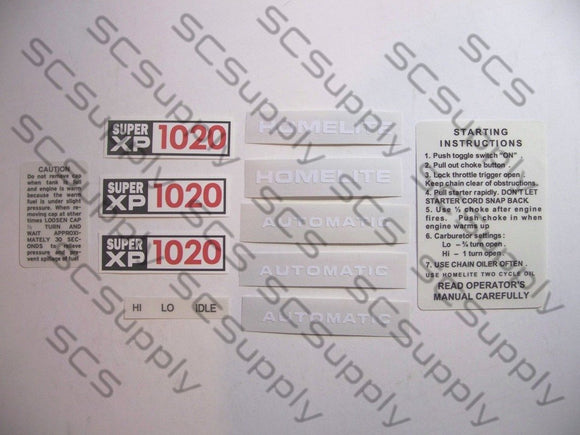This is a color photograph of various paper labels and stickers intended for a mechanical object, all arranged on a white surface. On the far left, there is a caution label with blurry text beneath the word "Caution". Next to it, there are three labels that say "Super XP 1020" in white on a red background. Below these, one label reads "H-I-L-O, Idle". In the central part of the image, there are two labels saying "Home Light" or "H-O-M-E-L-I-T-E". Adjacent to them, there are three labels reading "Automatic". On the right side, there is a detailed label titled "Starting Instructions" with steps for operating the machinery, including instructions for the choke, throttle, and carburetor settings, and a warning to use chain oil frequently, specifically Home Light II Cycle Oil, while emphasizing reading the operator's manual carefully. The entire photograph, which is rectangular in shape, has a watermark that reads "SCS Supply" repeated throughout the image.